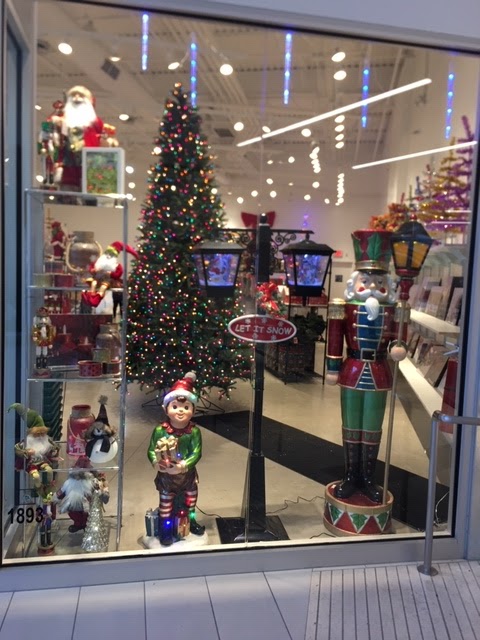This image captures a festive storefront display, likely situated indoors in a mall-like environment. The front of the store features a large glass window, making the dazzling array of Christmas decorations highly visible. Dominating the background is a brightly lit Christmas tree adorned with multicolored lights in red, green, and yellow. Prominently positioned in the forefront is a life-sized nutcracker statue, decked out in green pants and a red vest, and holding a golden streetlamp. To its left stands an elf figurine, dressed in a red Santa cap and green shirt, clutching a stack of gifts with more scattered at its feet.

Central to the display is a metal light pole with a festive red sign that reads "Let it Snow," surrounded by snowflake graphics. Additional Christmas decorations, such as Santa figures and gnomes, are arranged across various shelves and a glass counter cabinet. The scene is further enriched by reflections of twinkling lights in the glass and an exit sign visible deeper within the store, hinting at more holiday-themed merchandise like picture frames and additional Christmas trees. White tiling and a white wall frame the festive display, encapsulating the holiday spirit.